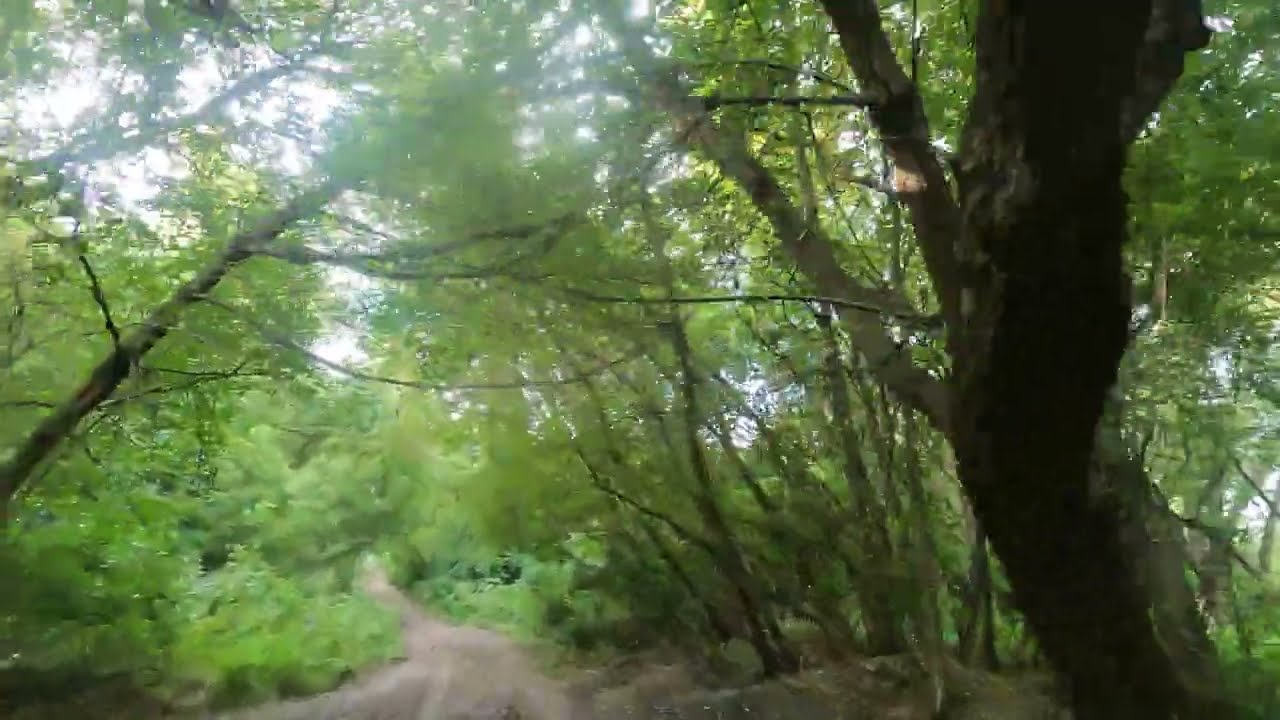A slightly blurred, horizontal rectangular image captures a serene dirt path winding through a lush, green forest. The path, about four feet wide and unpaved, is nestled between a dense array of trees and bushes, with greenery dominating the scene. The surrounding trees arch over the path, creating a natural canopy that blocks portions of the sunlight, contributing to the forest's tranquil ambiance. Bright green leaves, bushes, grasses, and weeds line the sides of the path, reinforcing the vivid green palette. A significant tree trunk is prominently visible on the right side of the image, extending from the bottom to the top, enhancing the sense of depth. Above the trees, patches of a partly cloudy sky peek through, adding subtle hints of light blue and white to the composition. The scene, devoid of people, animals, or vehicles, suggests a peaceful, late spring or summer setting. The image, with its soft focus, accentuates the lushness and tranquility of this woodland retreat.